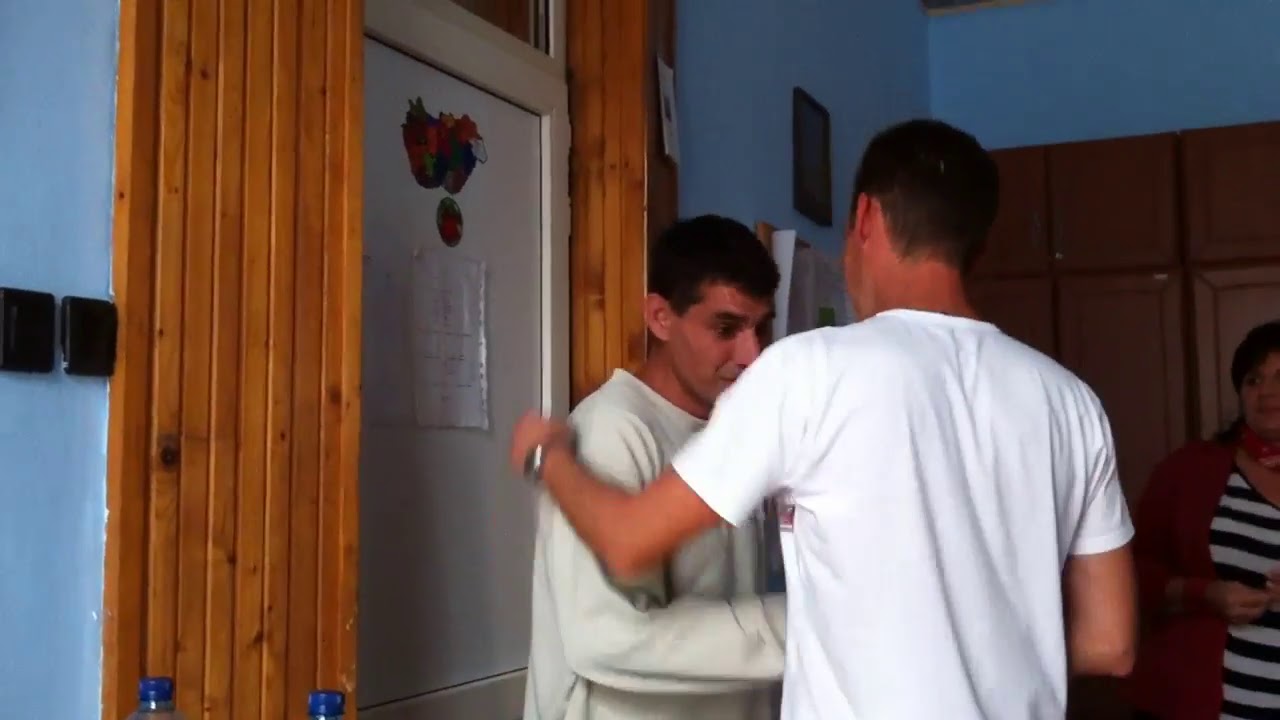In a room with blue walls and wooden cabinets, two men are caught in an intimate moment. The man on the left, wearing a white long-sleeve shirt, appears somber as he gazes downward, his eyes widened with a hint of sadness. The other man, standing with his back to the camera, has his arm around his companion’s shoulder, and is clad in a white t-shirt. Behind them stands a middle-aged woman with short dark hair, attentively watching the interaction. She’s dressed in a red sweater over a striped shirt. The setting includes a white door adorned with a multi-colored emblem and a piece of paper, flanked by wooden panels. The scene suggests a deep, emotional exchange, as the woman’s concerned gaze adds weight to the moment.